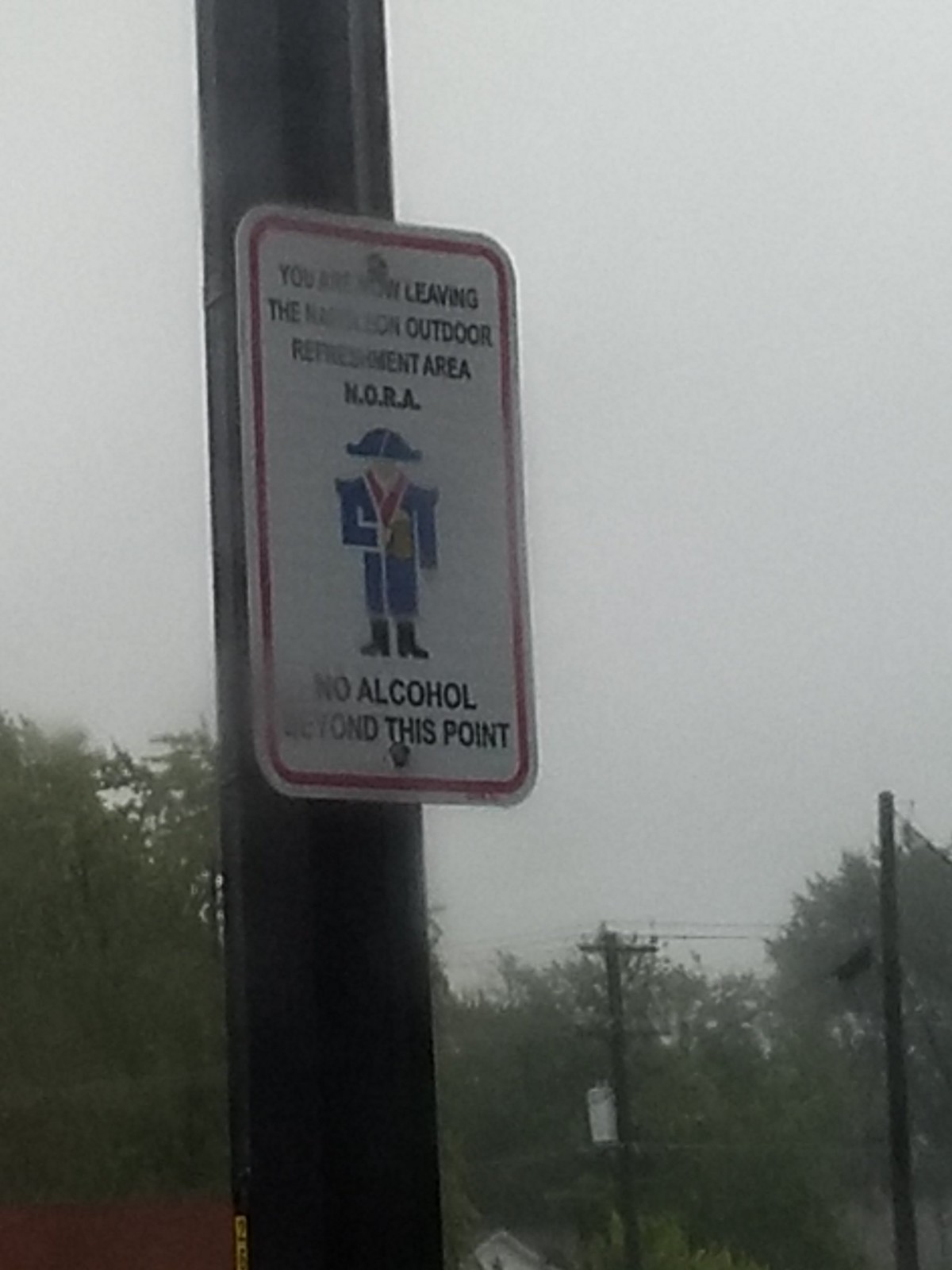This photograph, taken on a rainy, overcast day through a smudged or water-streaked glass, captures the scene from a slightly upward angle, focusing on a large, thick brown wooden pole centrally positioned. Attached to this pole is a rectangular white sign with a thin red border, fastened by two rivets at the top and bottom. The sign's black text partly reads "You are now leaving the [obscured] outdoor refreshment area, N.O.R.A.," alongside a simple cartoon-like soldier wearing a blue uniform and an old sailor's hat, holding a beer across his chest. At the bottom of the sign, it declares, "No alcohol beyond this point." The background is populated with large buildings, green trees, red fencing, and additional electricity and telephone poles connected by visible wires, all beneath a gloomy gray sky.